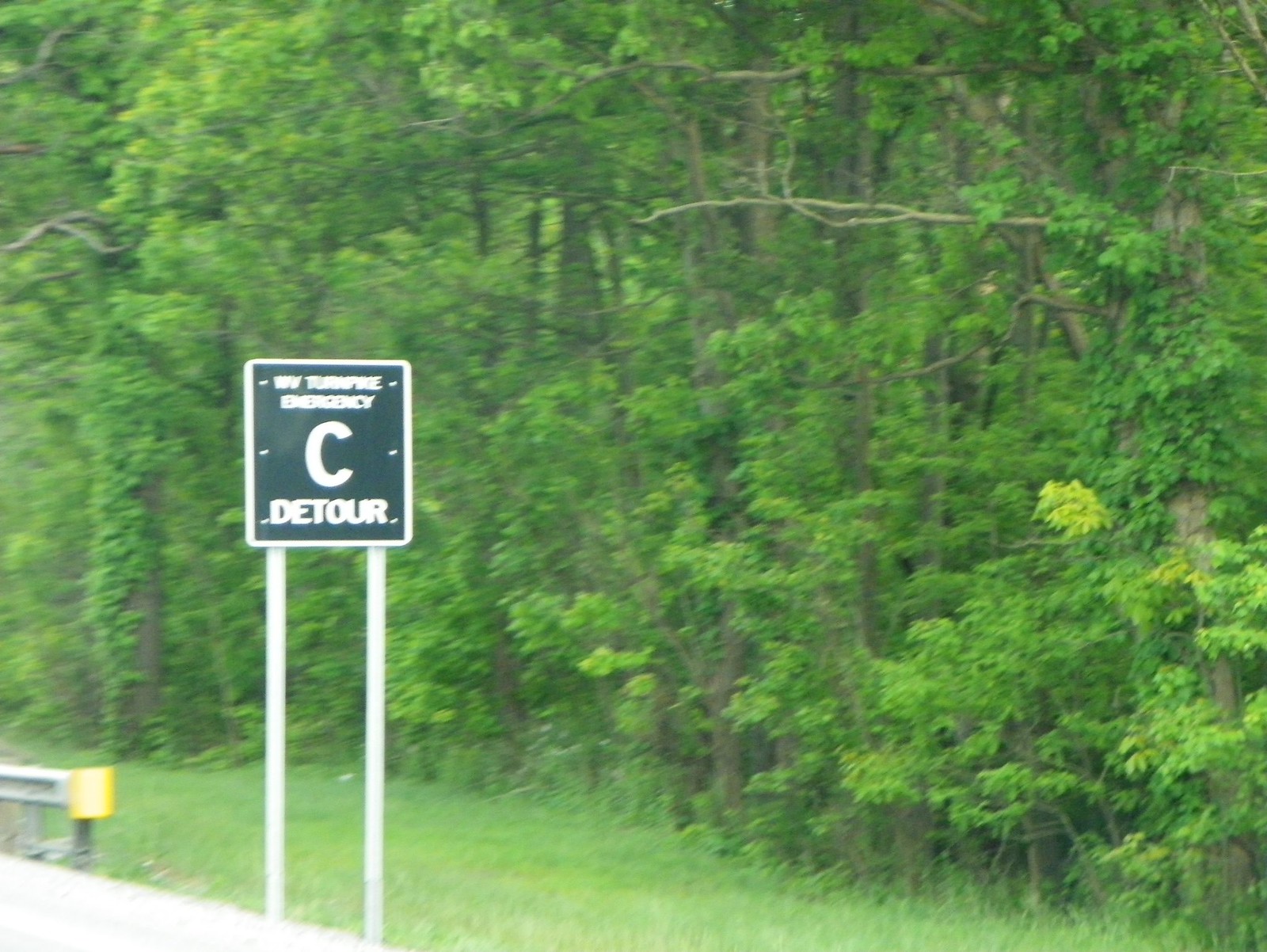This image captures a verdant roadside scene, likely taken from a car window in landscape orientation. Dominating the right side of the photograph is a dense, green forest with various trees, leafy branches, and new spring growth. The forest floor is adorned with tall, green grass. In the bottom left corner, a grey guardrail with a yellow reflective tip is visible, along with a small white triangle indicating the edge of the pavement.

Prominently featured slightly to the left of the image center are two light grey metal poles supporting a square, dark-colored road sign with white lettering. The sign, partially obscured and slightly blurred, reads "C Detour" and references an emergency route related to the turnpike. The exact wording above "C Detour" runs “New Hampshire Emergency.” The sign also has white dots decorating its sides. This detailed snapshot vividly depicts a lush, rainy spring setting.